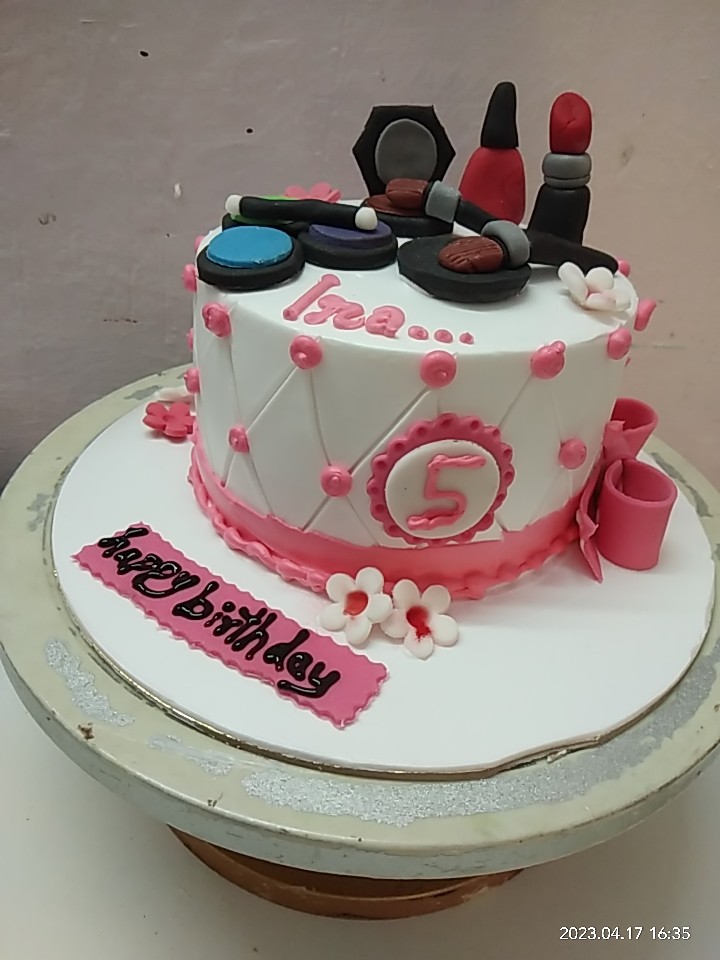This close-up photograph features a meticulously decorated one-tier birthday cake set against a pinkish-white wall. The cake, displayed on a white circular cake base, is exquisitely adorned with fondant and icing details. The lower portion of the cake showcases a pink rectangular fondant banner with little teeth cut out, enscribed with "Happy Birthday" in black cursive icing. The cake sits on a beige-tan silver platter and is bordered with a variety of fondant decorations. 

White fondant flowers with pink painted interiors embellish the side, accompanied by a pink flower on the left and another white flower, partly cut off by the photograph's angle. A bow fashioned from fondant appears on the right side, created with cylinders and additional fondant pieces. Pink fondant circles and an intricate embroidered fondant pattern encircle the cake, transitioning from flat to dotted lines. The inscription "IRA..." in pink fondant is present near the cake's base.

The top of the cake hosts an array of fondant pieces mimicking makeup items: black fondant circles topped with blue, purple, and lime green fondant, presumably representing eye shadows or foundation. There are cylindrical fondant brushes, one lying on a black fondant piece and the other on a brown one, with gray fondant mimicking metallic parts. A black fondant piece simulates a standing mirror with a gray interior, and adjacent to these are two objects resembling a red nail polish bottle with a black tapered lid and a black cylindrical piece topped with red fondant, likely representing red lipstick.

A prominent white fondant circle near the cake's middle features a pink "5" and is embellished with gilded icing around its perimeter. At the bottom corner of the picture, a timestamp reads "2023-04-17 16:35" in military time.